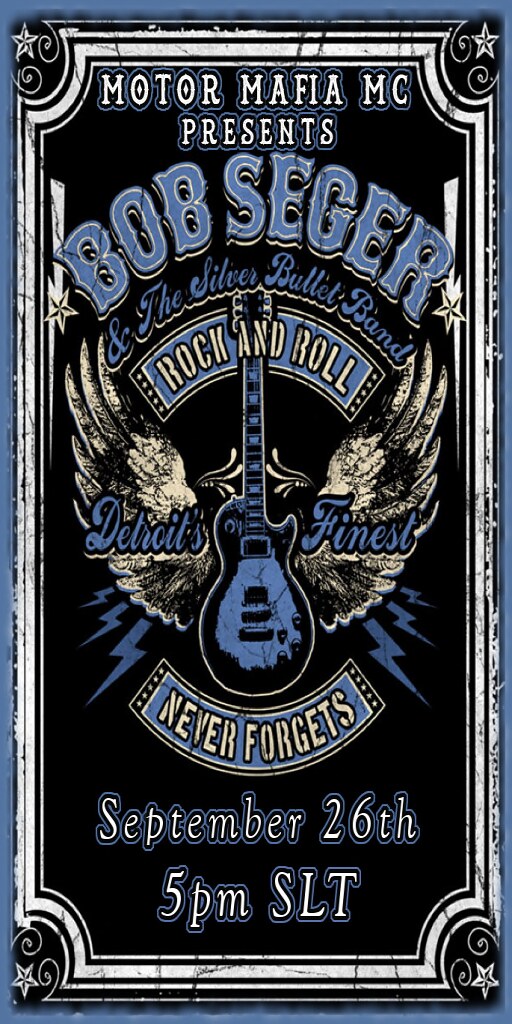This event poster features a striking, intricate design that commands attention. The border of the tall, rectangular poster is a solid, blue line framing an ornate white line with black stars in each corner, creating a sophisticated and eye-catching frame. Inside, the center of the poster is dominated by a solid black background adorned with various text and graphics.

At the very top, in an elegant white font bordered by black, it reads "Motor Mafia MC Presents". Below this, curved in a semicircle, "Bob Seger and the Silver Bullet Band" is prominently displayed in a bold blue font with white and black borders. A blue banner beneath this features the words "Rock and Row" in a white stenciled style font.

Central to the design is an imposing blue acoustic guitar with a white border, oriented with its neck pointing straight up. From either side of the guitar, white wings spread out, adding a dramatic, almost angelic element to the visual. In addition, the wings bear the phrase "Detroit's Finest," and below the guitar, lightning strikes and the phrase "Never Forgets" contribute to the dynamic energy of the poster. 

The poster further details the event date, "September 26th," and the time, "5 p.m. SLT," ensuring that all essential information is clearly communicated amid the visually rich backdrop.